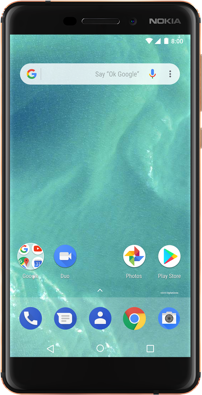This image depicts a highly pixelated and grainy compressed mock-up of a Nokia smartphone. The Nokia logo is prominently displayed in the top right corner of the device, situated on a curved bevel that simulates a glimmer of shine. The screen features a top-down image of an ocean, with a Google search bar at the very top. Within this bar, you can see the iconic "G" on the left side followed by the text "OK Google" next to a microphone icon.

At the top of the screen, there's information about the network signal bars, battery life, and the time, which is shown as 8:00. Moving down, there are four recent icons just above the standard five permanent icons. These recent icons represent various Google applications: Google itself, Duo (depicted by a movie camera icon), Photos (represented by a pinwheel icon), and the Google Play Store (highlighted with a triangular logo).

The screen is partially overlaid by a translucent white gradient, possibly around 30% transparency, which lightly obscures the image beneath. The five permanent icons at the bottom include a phone icon, a text speech bubble (likely for messaging), a profile button, the Chrome browser icon, and a camera icon. Below these, the navigation bar features the traditional Android buttons: a back arrow (triangle), a home button (circle), and the recent apps button (square).